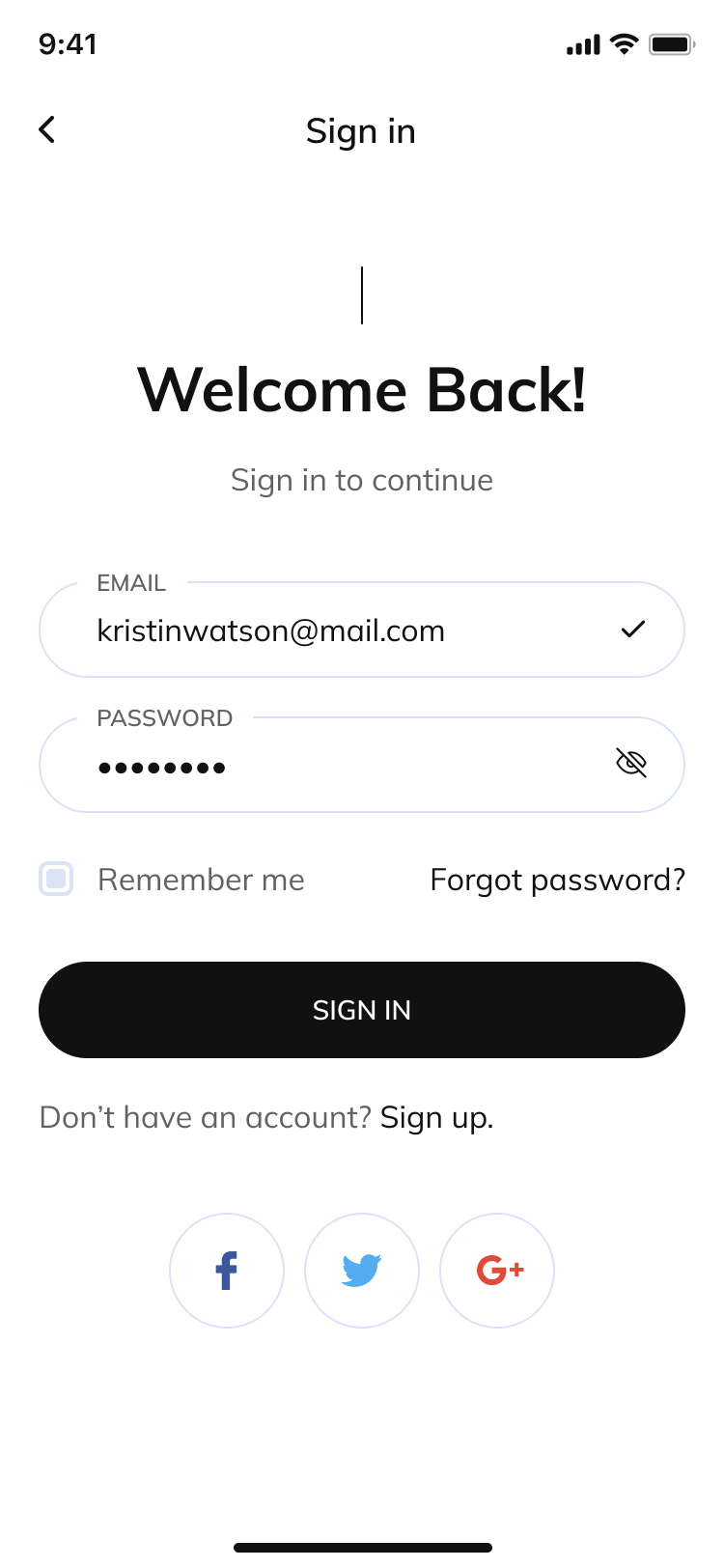The image displays a login screen on an unidentified device. 

At the very top, there is a status bar indicating it is 9:41 AM. The status bar includes icons for Wi-Fi (four bars), cellular signal strength (four bars), and battery status (fully charged). Below this, a progress bar is positioned at the halfway mark.

Beneath the status bar, aligned to the left, is a leftward-pointing arrow next to the text "Sign In." A large section of blank space follows before reaching a welcoming message in bold black font reading "Welcome Back!" Below this, in a lighter gray font, is the prompt "Sign in to continue."

The main login fields are centered on the interface. First, an elongated oval field labeled "Email" displays an example email address, "kristinwatsonatmail.com," next to a check mark indicating a valid entry. Underneath is another elongated oval labeled "Password," filled with dots representing hidden characters. An icon of an eye with a slash through it indicates the obscured password. 

Below the password field, the options "Remember me" are displayed, alongside the "Forgot password?" link. The sign-in button, a dark black oval with white text, offers the prompt "Sign In."

At the bottom of the screen, a message reads "Don't have an account? Sign Up," encouraging new user registration. Finally, icons for Facebook, Twitter, and Google Plus are aligned at the very bottom, signifying alternative login methods.